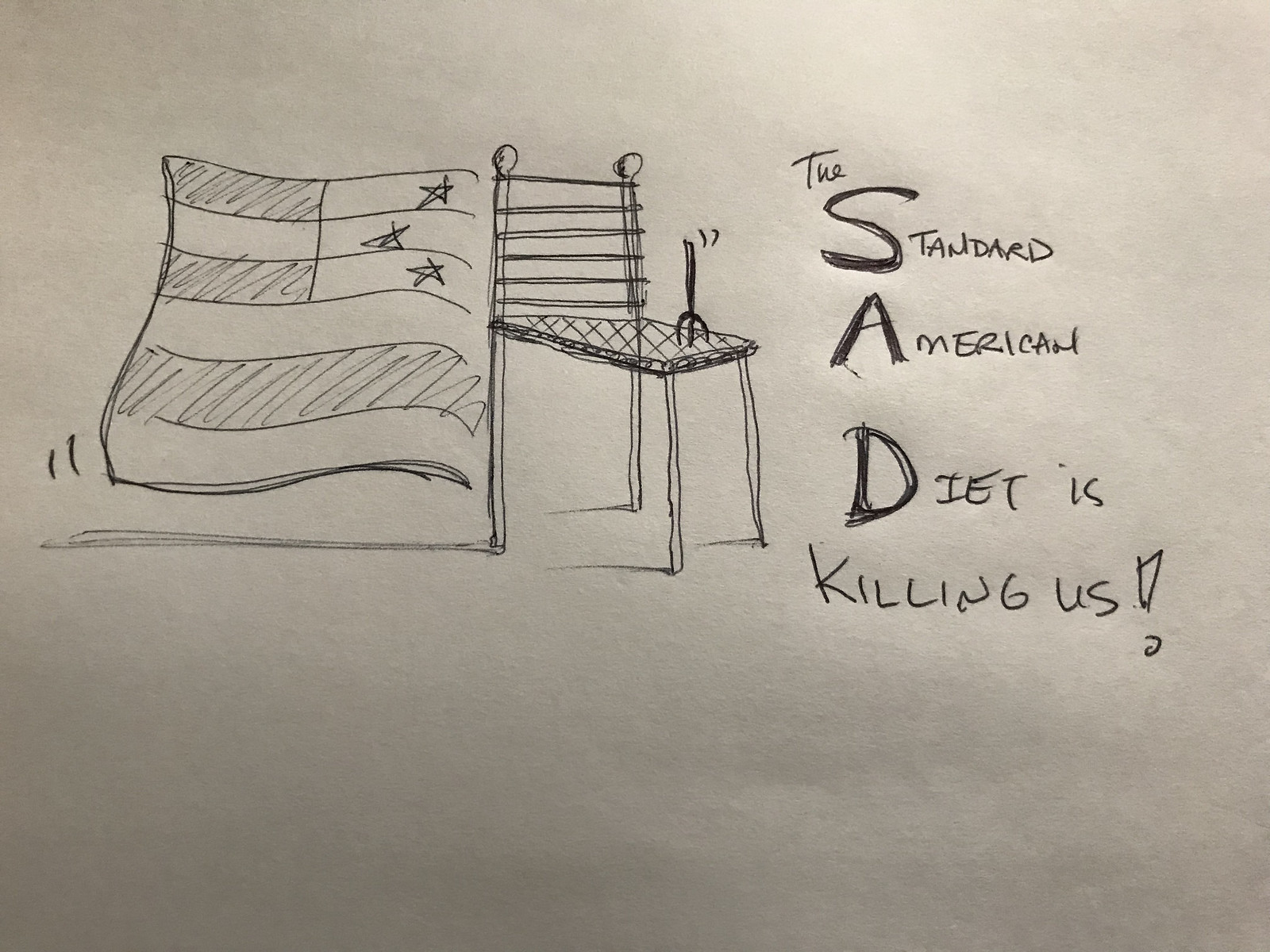A detailed black-and-white hand sketch depicts a simple four-legged kitchen chair. Intriguingly, an upside-down tiny pitchfork is embedded into the seat of the chair. Attached to the chair is a waving flag, which, despite the absence of color, is identifiable by its stars and stripes as the American flag. Handwritten on the right side of the chair, in small letters, is the word "the," followed prominently by the letters "S-A-D," forming the word "sad." Adjacent to this, a larger inscription reads: "standard American diet is killing us!" punctuated emphatically.